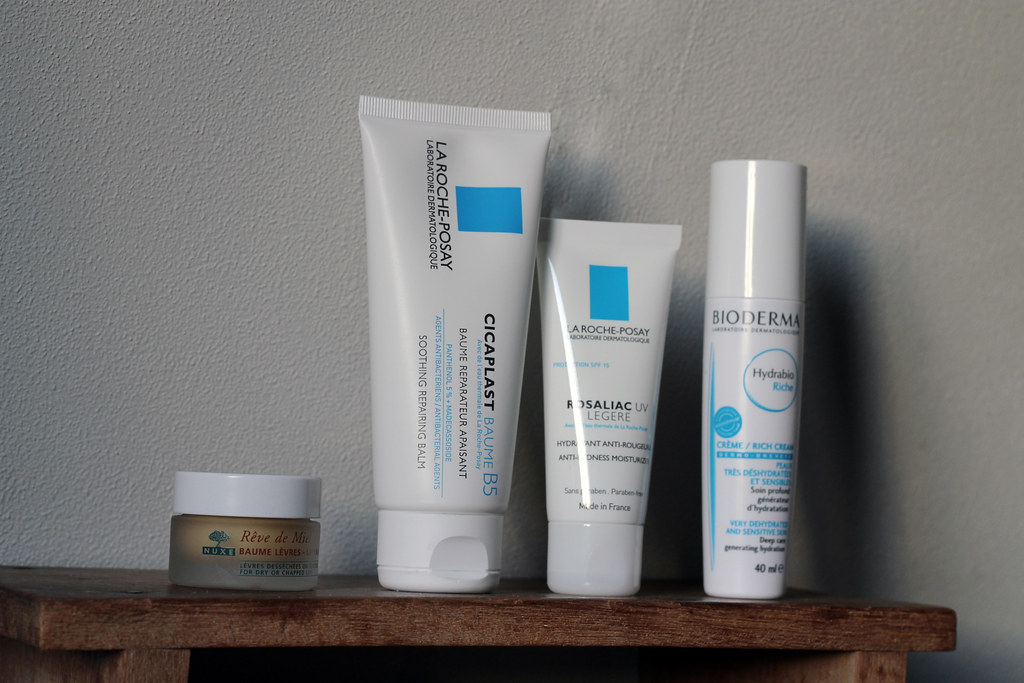In this image, taken inside a somewhat modest bedroom, we can observe a white wall with a rough, uneven texture suggesting a less-than-perfect paint job. At the bottom of the image, a dark brown shelf, with a slightly lighter brown trim on the sides, spans horizontally across the frame. Resting on this shelf are four personal care products arranged in a row. 

Starting from the left, there is a small bottle with a prominent white cap. The label on this bottle reads "Rev de M.I.C." in red text, with additional text below that states "Bomb Levis." 

Next to this, we have a larger, cylindrical item, possibly a spray or tube, featuring a clean white design. The top of this object bears the brand name "La Roche-Posay," and towards the bottom, it reads "Cicaplast Baume B5."

Continuing to the right, there is a smaller product from the same brand, "La Roche-Posay." Its label indicates it is "Rosaliac UV Legere."

The last item on the far right is another product bearing the brand "Bioderma," with its label indicating it is from the "Hydrabio" range. Each item appears to be skincare and haircare-related, neatly lined up on the dark brown shelf against the textured white wall.